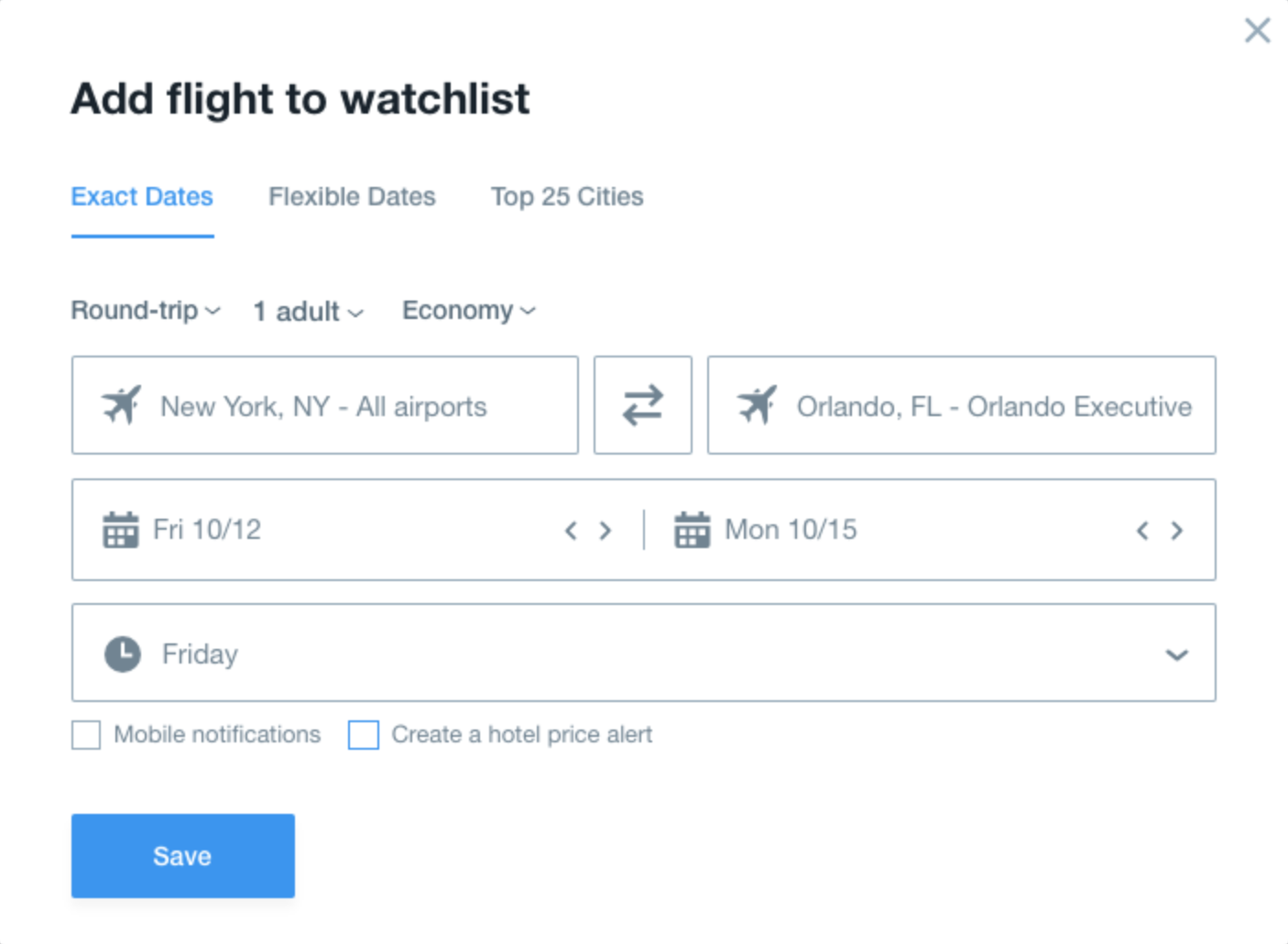**Screenshot Details of Flight Watchlist Addition**

The image is a horizontally rectangular screenshot on a white background. 

**Top Section:**
- **Top Left Corner:** Enlarged, bold text reading "ADD FLIGHT TO WATCHLIST."
- **Top Right Corner:** An "X" button to close the window.

**Selection Options:**
- Directly beneath the heading are three selectable options:
  - **Exact Dates**
  - **Flexible Dates**
  - **Top 25 Cities**

**Trip Details:**
- Below the selection options are dropdown menus specifying:
  - **Trip Type:** ROUND TRIP
  - **Number of People:** ONE ADULT
  - **Class:** ECONOMY

**Location Fields:**
- Next are three side-by-side input fields:
  - **Origin:** NEW YORK, NEW YORK, ALL AIRPORTS
  - A reverse button
  - **Destination:** ORLANDO, FLORIDA, ORLANDO EXECUTIVE

**Date Selection:**
- **Departure and Return Dates:** Friday 10-12, Monday 10-15
- A dropdown menu for selecting the specific **day** starting with Friday.

**Notification Options:**
- Two checkbox options beneath the date selection:
  - **Mobile Notifications:** Unchecked and grayed out
  - **Create a Hotel Price Alert:** Unchecked and outlined in blue

**Save Button:**
- A blue "SAVE" button located in the bottom left corner.